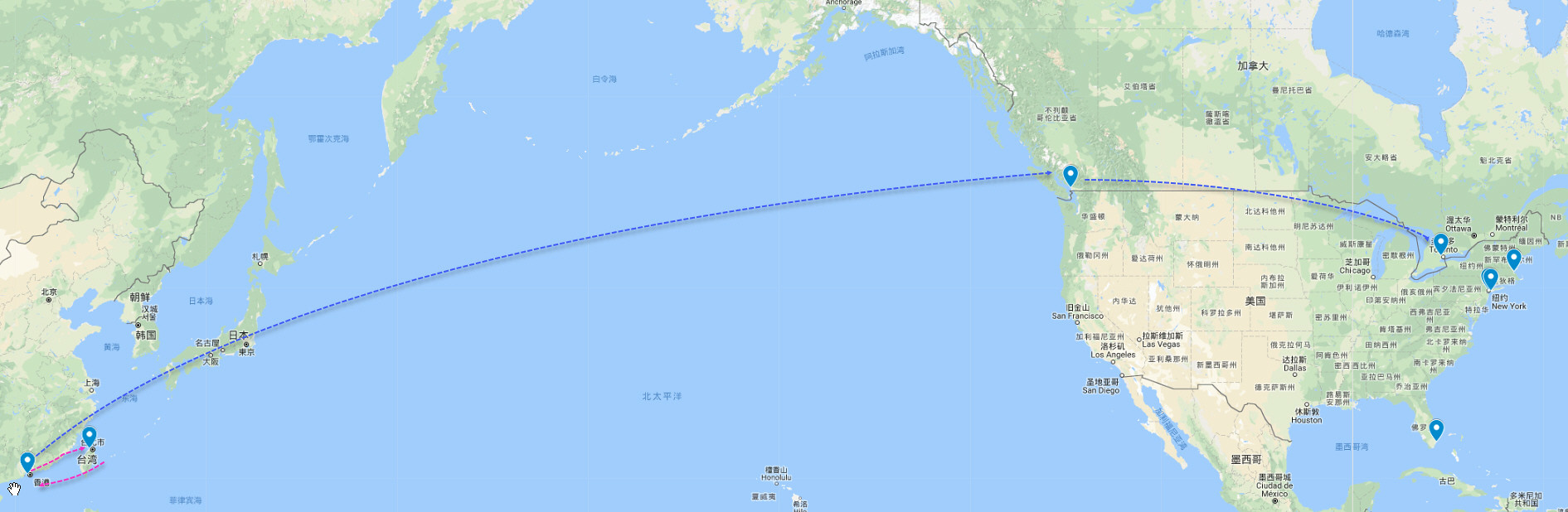This image is a detailed screenshot of a Google Maps flight route, heavily annotated in Chinese characters. The map covers parts of the Northern Hemisphere, including regions such as China, Western Russia, Japan on the left side, and the contiguous United States, southern Canada, and northeastern Mexico on the right. Clearly visible is an arcing, blue-dashed line representing flight paths. The line starts between two major cities in China, possibly Beijing and Shanghai, traverses the Pacific Ocean, and stops in Vancouver. It then continues across North America touching down in Toronto, and possibly routes to New York or nearby cities like Boston, Massachusetts, or a location in Florida. The specific map pins and connecting lines illustrate a detailed travel itinerary with multiple international stops.